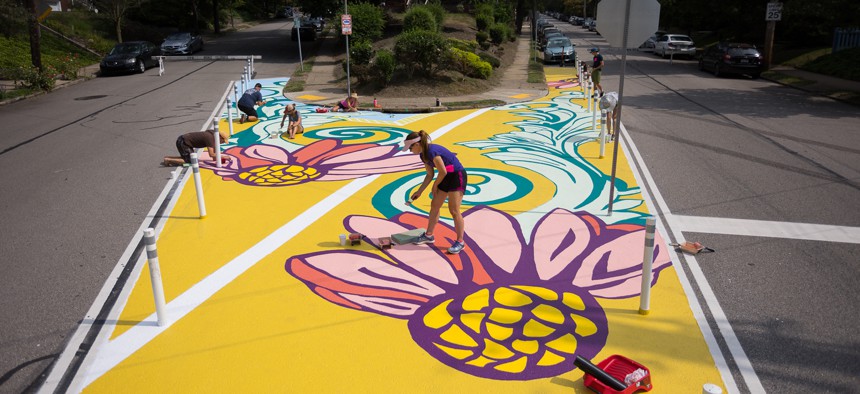In this vibrant and bustling urban scene, artists are diligently at work painting a stunning mural on the asphalt of a triangular median area set at the fork of a city street. Surrounded by a backdrop of meticulously planted shrubs and a curving sidewalk, the artists bring the median to life with intricate, bright floral patterns. The mural features a radiant sunflower-yellow background adorned with captivating white stripes and swirly blue and green accents. Central to the artwork is a series of large, pink and peach flowers with purple centers ringed with yellow, resembling a burst of floral exuberance amidst the urban setting.

In the foreground, a woman wearing a purple shirt, black shorts accented with hot pink, and a white headband, carefully stoops over her section of the mural, her red paint tray with tools beside her. This scene captures her meticulously painting the vibrant petals of the flower. Surrounding her, other artists—both men and women dressed in shorts and t-shirts, some wearing sun visors—are similarly engrossed in their work, either on their knees or lying on the ground to reach the mural’s extensive surface.

The median, demarcated by white metal poles, extends from a hillside of shrubbery and features the identical floral and aquatic patterns repeated in varying configurations. The scene is bathed in bright sunlight, enhancing the vivid colors of the mural and highlighting the collective artistic effort transforming an ordinary piece of the cityscape into a visually stunning masterpiece.